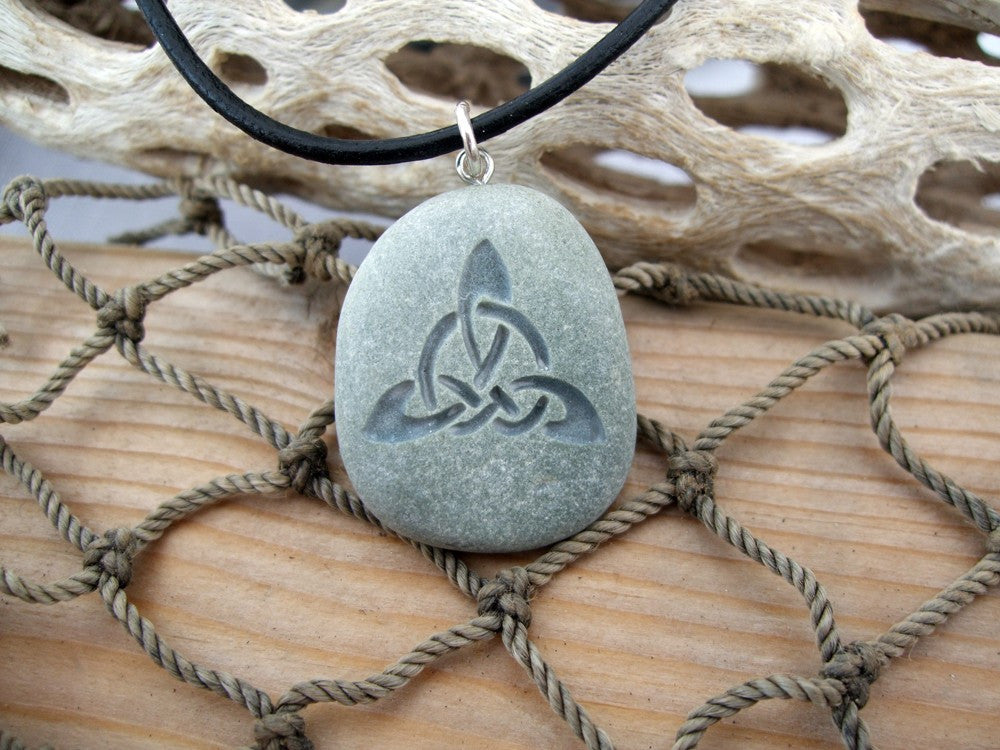The image showcases a close-up of a necklace prominently featuring a pendant. The necklace appears to be crafted from a leather-look or PVC cord, fitted with a silver-tone jump ring that secures the pendant. The pendant itself is made from a gray stone or stone-like clay and intricately etched with a Celtic cross pattern. Surrounding the central cross are additional concentric rings and triangular shapes, radiating out from the center of the design. The necklace is displayed on a light brown woodgrain surface, partially covered by a grayish-brown fishnet rope, contributing to a beach-inspired aesthetic. The overall color palette of the image includes tones of black, silver, brown, and bluish-gray, and the background is somewhat hazy, evoking an overcast, possibly beach-like setting.